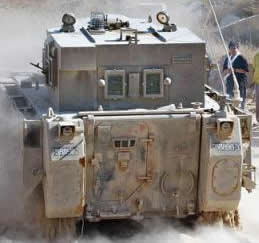This is a color photograph capturing the back of an old, rusted, armored military vehicle, distinguished by its robust, rectangular structure and dusty environment. The vehicle's bottom level is grayish-pink with rust and gray dirt, while the upper level is a dark, weathered gray. The back of the vehicle features a flat, square metal panel with protruding rectangular shapes on both sides. The vehicle appears to be moving away, kicking up a significant amount of dust, partially obscuring its lower section and contributing to the dusty atmosphere. There are two rectangular windows on the second level, one of which has a gun protruding from it. The top of the vehicle houses some black objects that might be part of its equipment. On the top right side of the image, a blurred figure, likely a person in a black shirt with a white neckline, stands nearby. In the background, a child with tan skin and a towel around his neck is observing the vehicle. The overall backdrop is a grayish-white, further emphasizing the vehicle's rugged, battle-worn appearance.